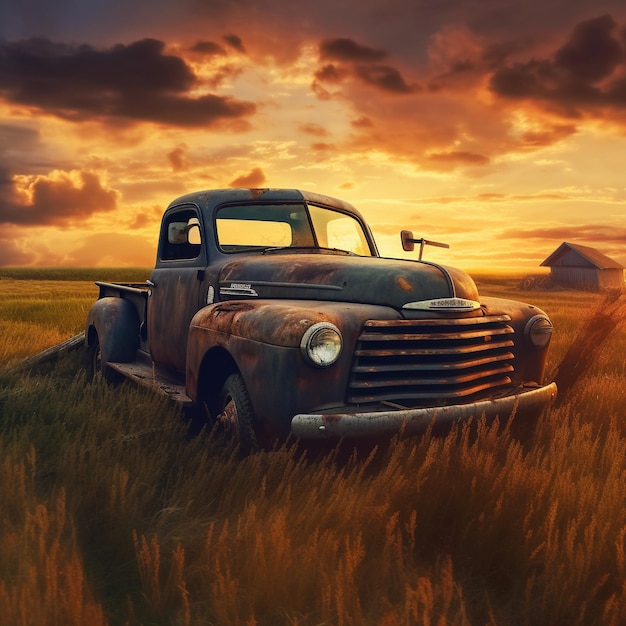This detailed illustration features a vintage, heavily rusted pickup truck, likely from the 1930s or 1940s, parked in the center of a field overgrown with tall, golden and green weeds, reminiscent of a meadow. The truck, with its gray, rust-speckled body, missing passenger-side window, large rearview mirrors, running board, and distinctive two-piece windshield, embodies a bygone era. Its chrome bumper contrasts with the dilapidated wheels that appear flat. The setting sun or rising dawn paints the sky in shades of orange, dark orange, and grayish blue, mirroring the hues of the dry grass below. To the right, a simple, nondescript barn or cabin stands, devoid of windows and doors, its straightforward structure contributing to the scene's nostalgic ambiance. The artistic style, whether painted traditionally or created digitally, aptly captures the serene yet desolate beauty of this rural landscape.